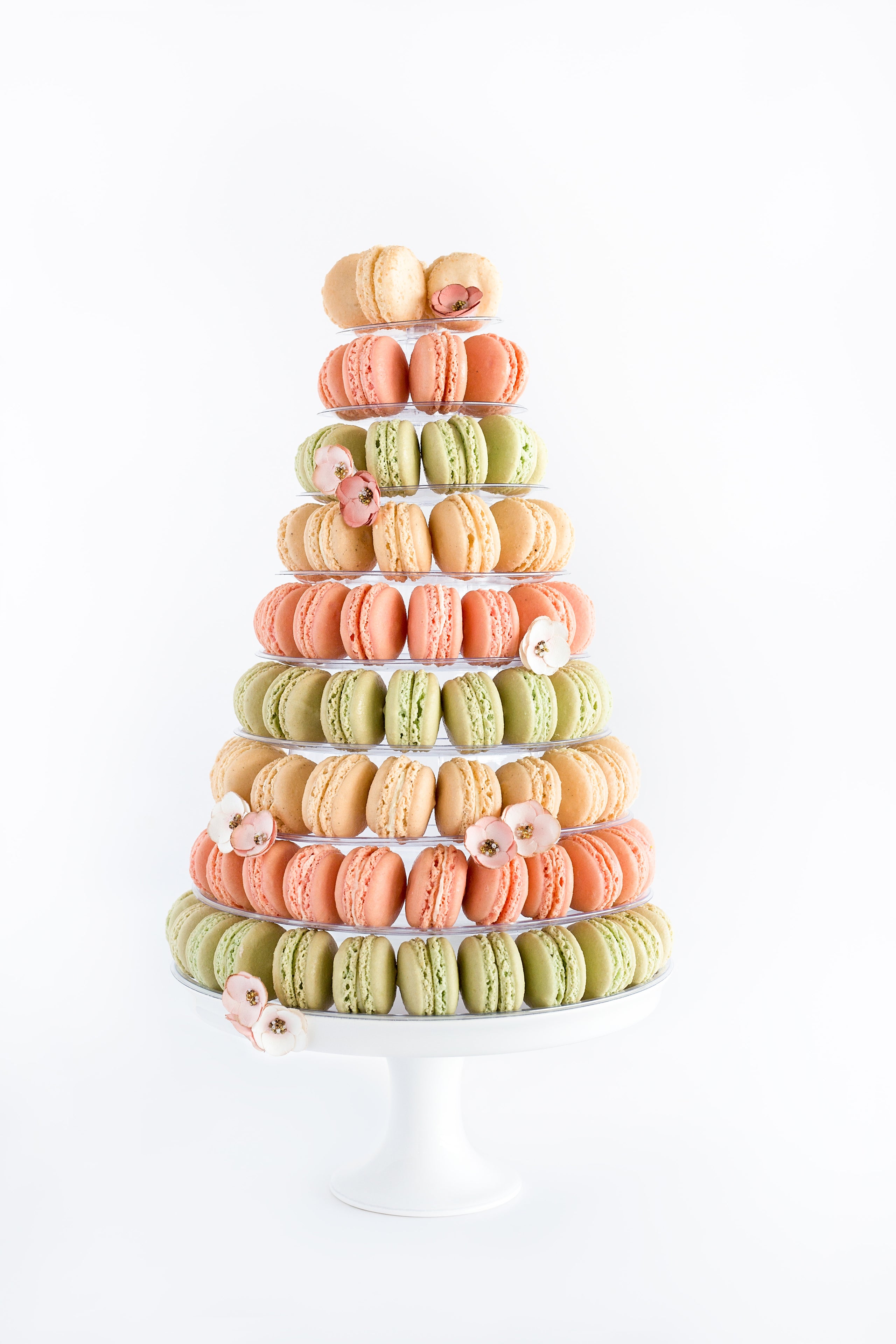The image showcases a tiered white stand that is structured to resemble a Christmas tree, featuring multiple layers of colorful macarons. The stand's design narrows from a broad base to a small top, giving it a conical, tree-like shape. The macarons are arranged in alternating colors of green, pink, and pale yellow (or a matcha green, soft red-pink, and light beige), with each layer becoming progressively smaller as they ascend the stand. The macarons are placed on their sides, revealing the cream filling. Scattered throughout the layers, pink flowers add decorative flair, with one flower at the top row, and more flowers interspersed at various points below. The entire setup is placed on a white porcelain dish, against a stark white background, emphasizing the pastel hues and the tree-like structure of the macarons.